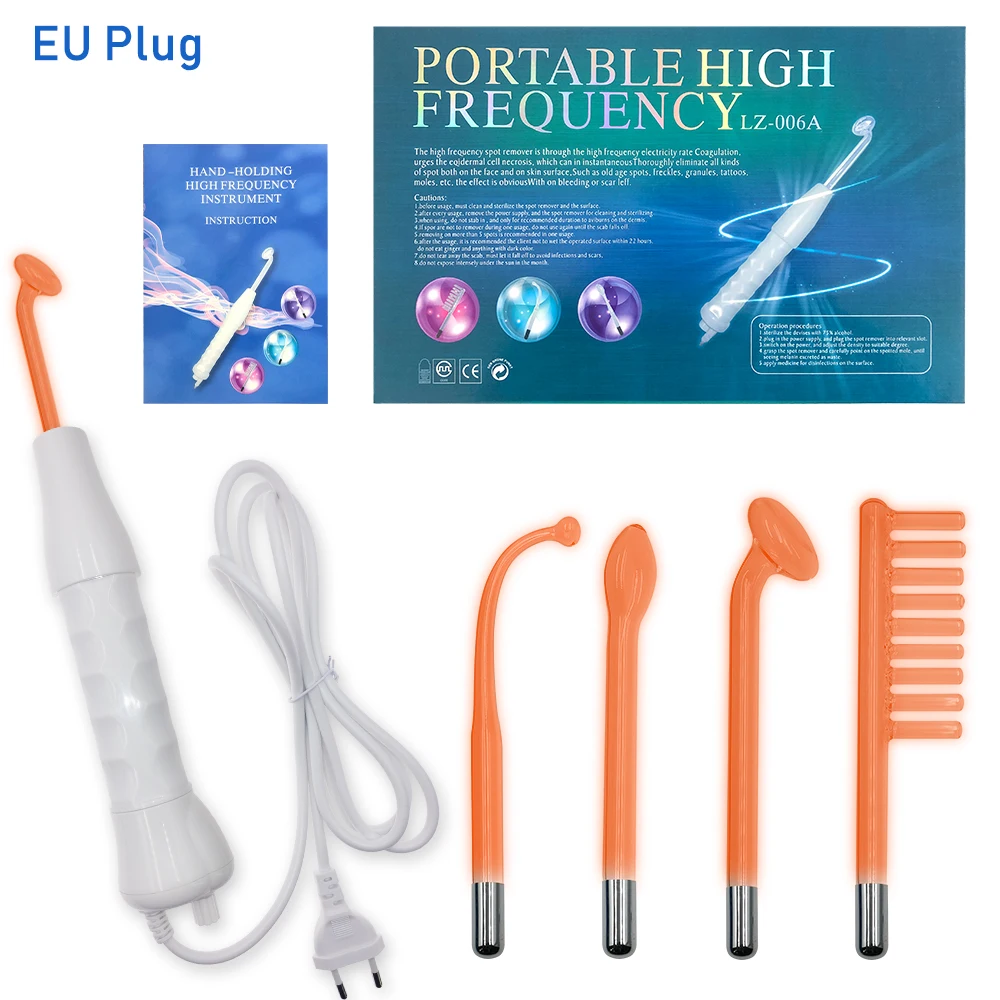The image shows a portable high-frequency instrument, prominently displaying the European plug compatibility in the top left corner. At the top, there are two descriptive boxes: the smaller blue box on the left labeled "Hand Holding High Frequency Instrument Instruction" and the larger turquoise box labeled "Portable High Frequency LZ-006A." The device itself, located in the bottom left of the image, consists of a white handle and a white cord, with an orange rod attachment at the top. The bottom right features various interchangeable attachments, including a fine point, a broader point, and a brush or comb-like attachment, all in bright orange with metal poles that fit into the base of the white handle.